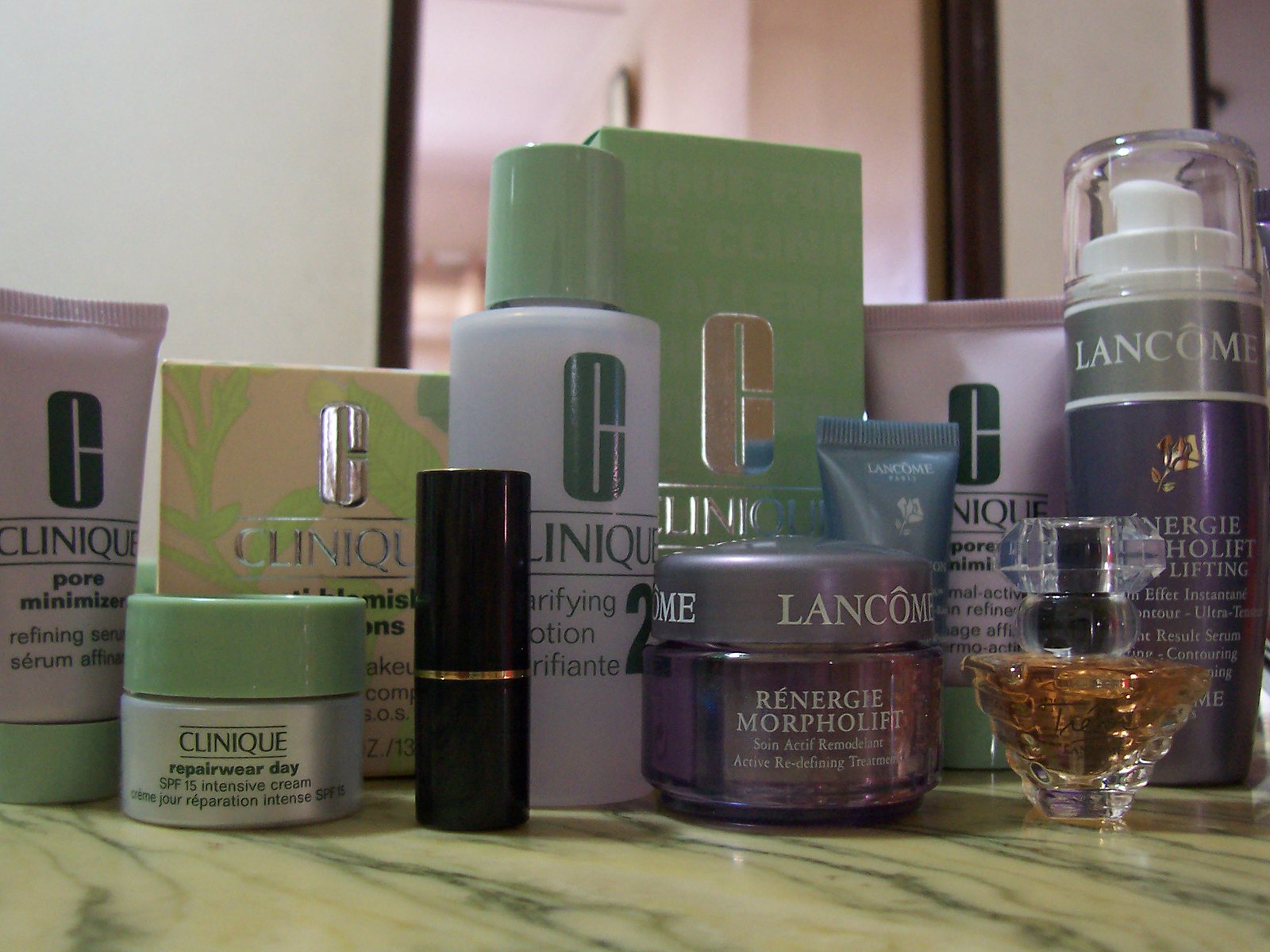This color photograph captures a close-up view of a makeup counter, likely within a department store, given the sophisticated arrangement and variety of high-end products displayed. The surface of the counter is made of polished marble, enhancing the elegance of the scene. Dominating the counter are products from Clinique and Lancôme, meticulously organized in neat rows.

Starting from the left, the first product is a Clinique Pore Minimizer, easily recognizable by its iconic soft green squeeze tube and cap, standing upright. Next is a small Clinique Repairwear Day SPF 15 Intensive Cream, housed in a clear glass jar with a green screw-on top, designed for easy application and travel convenience. Partially obscured behind this jar is a packet of Clinique products, though the exact contents remain indistinguishable.

Further along the counter, a striking black lipstick case with a gold band adds a touch of classic sophistication to the display. Adjacent to this is a bottle of Clinique Clarifying Lotion, marked as step two in their skincare routine, featuring a transparent bottle capped with the signature Clinique green.

Behind these products, a Clinique green box embossed with the silver Clinique "C" logo stands, partially hidden by other items in the foreground. Adding to the collection is a small, lavender-hued jar of Lancôme Renergie Morpholift, an upscale face cream, accompanied by a coordinating small lavender-blue squeeze tube with a delicate calla lily design.

Reiterating the visibility of Clinique’s signature product line, another Clinique Pore Minimizer appears identical to the one on the far left. Following this is a sleek, tall Lancôme bottle with a clear plastic cap, dispensing product via a press-down mechanism. It is labeled with references to energy and lifting, suggesting an advanced serum or lotion.

Adding a final touch of luxury, there is a distinctive perfume bottle shaped like an upside-down Christmas tree. It contains a rich amber liquid and features a crystal-like top with a misting sprayer, ready to envelop the user in an elegant fragrance.

In the background, behind the counter, is what appears to be either a mirror or a window, contributing to the spacious and bright atmosphere typical of a well-appointed department store.